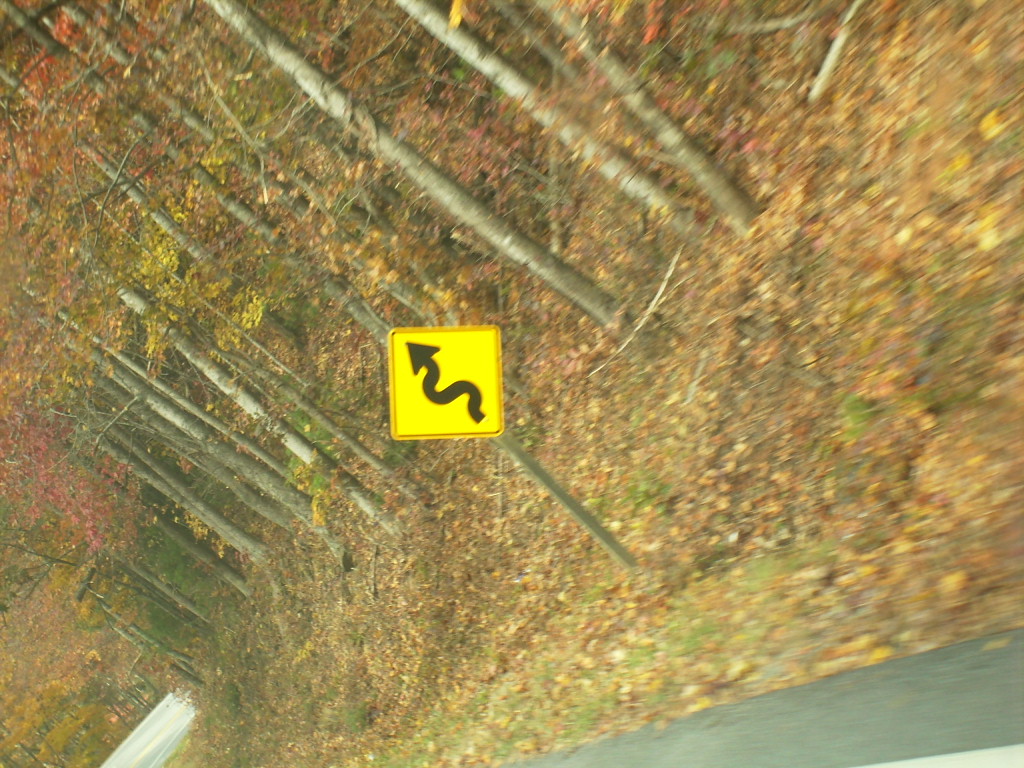The photograph captures an outdoor scene in what appears to be a forested, hilly area during the fall season. Dominating the image is a yellow diamond-shaped street sign, mounted approximately four feet high on a wooden post, with a squiggly black arrow indicating a curvy road ahead. The sign has hints of a red border. The bottom portion of the picture features a dark gray asphalt road bordered by light green grass interspersed with fallen red, orange, and brown leaves. The road curves, as suggested by the sign. The upper two-thirds of the image showcases a dense forest of trees with trunks of gray and a mix of foliage in various stages of autumnal transformation, displaying hues of dark red, yellow-green, orange, and light brown. Leaves are scattered on the ground, emphasizing the seasonal change. The overall scene presents a vivid impression of a winding roadway through a colorful, leaf-strewn forest in fall.